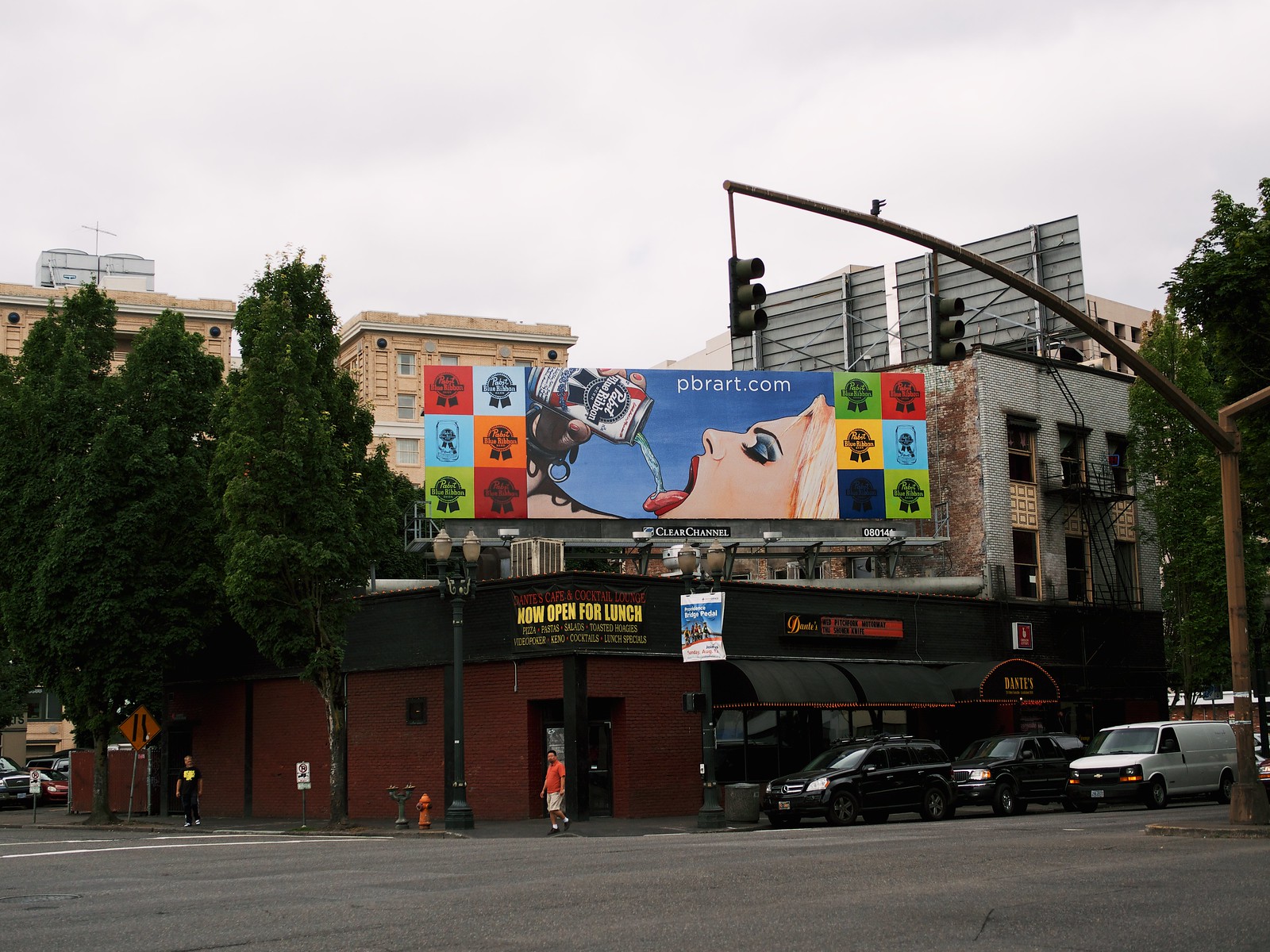The image depicts a bustling street corner dominated by a brick building with a striking facade in a 90-degree angle. The left side of the building is brick while the right side features black walls adorned with mood-lit awnings. At the center of the image, a prominent entrance to Dante's Cafe and Cocktail Lounge, marked by gold and red lettering, announces "Now Open for Lunch," though additional text is difficult to decipher. To the right of the entrance, there are three parked cars—two black and one white van. Two men, one in an orange shirt and gray shorts and the other in a black outfit, stand near the entrance, seemingly looking towards the camera. Above the cafe, a vibrant Pabst Blue Ribbon billboard in pop art style attracts attention. It features an array of colorful squares and a central image of a woman pouring beer into her mouth, flanked by the Pabst logo on both sides. The building is surrounded by several tall trees and, in the background, a few high-rise buildings and a clear blue sky complete the urban landscape. In the foreground, the street is busy with moving cars, a pedestrian walkway on the left, and a streetlight pole near the white van adding to the city vibe.